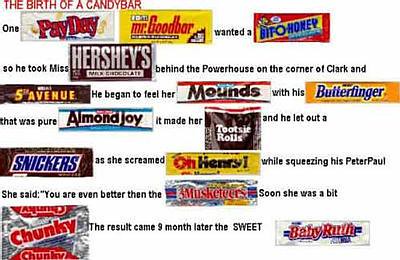The image, in landscape format and in color, presents a clever short story titled "The Birth of a Candy Bar" in vivid red block letters at the top. Though the photo is small and low-resolution, it intricately weaves images of various candy bars into the text, using their names to form a playful narrative. The tale begins with "One Payday Mr. Goodbar wanted a bit o' honey, so he took Miss Hershey’s behind the powerhouse on the corner of Clark and Fifth Avenue." The story continues with Mr. Goodbar exploring Miss Hershey’s “mounds with his butterfinger,” leading to a series of comic and risqué candy-themed double entendres involving Almond Joy, Tootsie Rolls, Snickers, and Oh Henry bars. The narrative humorously concludes with Miss Hershey becoming “a bit chunky” and giving birth to “the sweet Baby Ruth.” The photo cleverly uses the images of the candy bars, including Payday, Mr. Goodbar, Bit o' Honey, Hershey's, Fifth Avenue, Mounds, Butterfinger, Almond Joy, Tootsie Roll, Snickers, Oh Henry, Three Musketeers, Chunky, and Baby Ruth, to visually represent each candy name within the text.